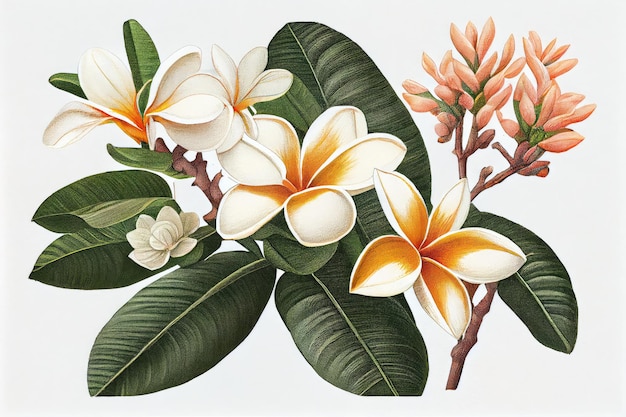This painting showcases a detailed depiction of a plant with a stark white backdrop that accentuates its vibrant elements. The foreground features a prominent brown branch that stretches from the bottom right corner towards the center, branching out to support lush, dark green, oval-shaped leaves. Alongside the leaves, there are beautiful flowers and buds. 

The composition includes a diagonal row of four large white flowers, each exhibiting goldish-brown streaks and fading to orange in the center, trailing from the top left down to the bottom right. Adjacent to this row, a smaller white flower with subtle hints of mint green adds variety to the floral arrangement. 

On the top right side, two smaller branches bear numerous pinkish-peach buds that haven’t yet opened, suggesting the imminent bloom of more flowers. Scattered among these buds, you can spot a few small spherical buds, hinting at future blossoms. The overall composition of green leaves and multi-hued flowers against the plain white background creates a vivid and detailed botanical illustration.